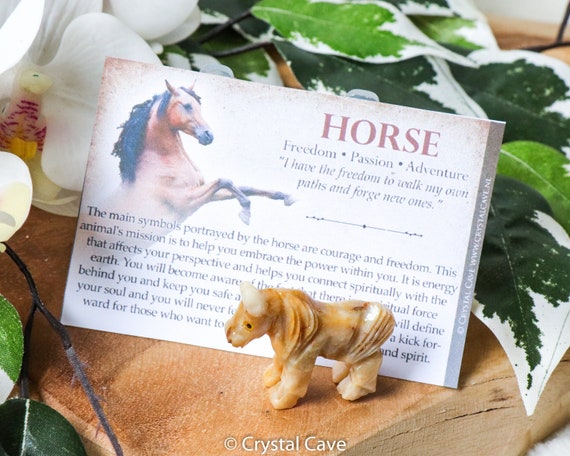This photograph showcases a decorative card with a central illustration of a horse rearing on its hind legs. The horse, depicted with a black mane and a caramel-colored coat, symbolizes themes of freedom, passion, and adventure. The card features text in burgundy and black fonts, reading: "Horse. Freedom, passion, adventure. I have the freedom to walk my own paths and forge new ones." Additional descriptive text in black font states: "The main symbols portrayed by the horse are courage and freedom. This animal's mission is to help you embrace the power within you. Its energy affects your perspective and helps you connect spiritually with the earth. You will become aware of the…" (the text is partially obscured).

The backdrop includes green plants with white outlines and delicate white flower petals. In the foreground, there is a small, decorative horse carving. At the bottom of the image, a white watermark reads "Crystal Cave," which matches the card's website URL, www.crystalcave.com.